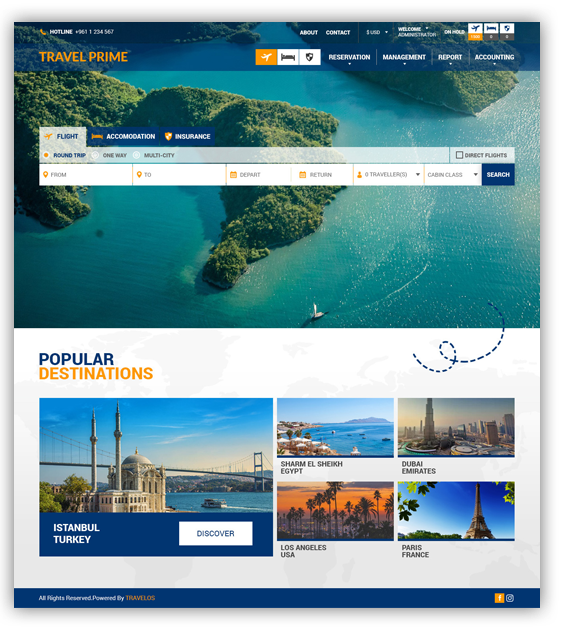**Detailed Caption:**

This image is a screenshot from the Travel Prime webpage. The website's name "Travel Prime" is prominently displayed in uppercase, orange letters on the top left side. Directly above the website name is a hotline number for customer inquiries. On the same row, there are several navigation tabs including "Flight" (highlighted in orange), "Hotel," and "Insurance," each with a white background except for the active one. Adjacent to these tabs are additional links titled "Reservation," "Management," "Report," and "Accounting."

The main visual of the webpage is a captivating background image of an island surrounded by clear, tranquil blue waters. Superimposed on this image is a functional chart with three tabs: "Flight," "Accommodation," and "Insurance." Under the "Flight" tab, users can choose from three options: "Round Trip," "One Way," and "Multi-City." The chart includes input fields for the departure and destination locations, departure and return dates, a section to specify the number of travelers and cabin class, and a blue search button. Additionally, there is a checkbox for selecting direct flights only.

At the bottom of the webpage, there is a section titled "Popular Destinations" showcasing enticing images of renowned travel spots around the globe. Featured destinations include Istanbul in Turkey, Sharm el Sheikh in Egypt, Los Angeles in the United States, Dubai in the United Arab Emirates, and Paris in France.